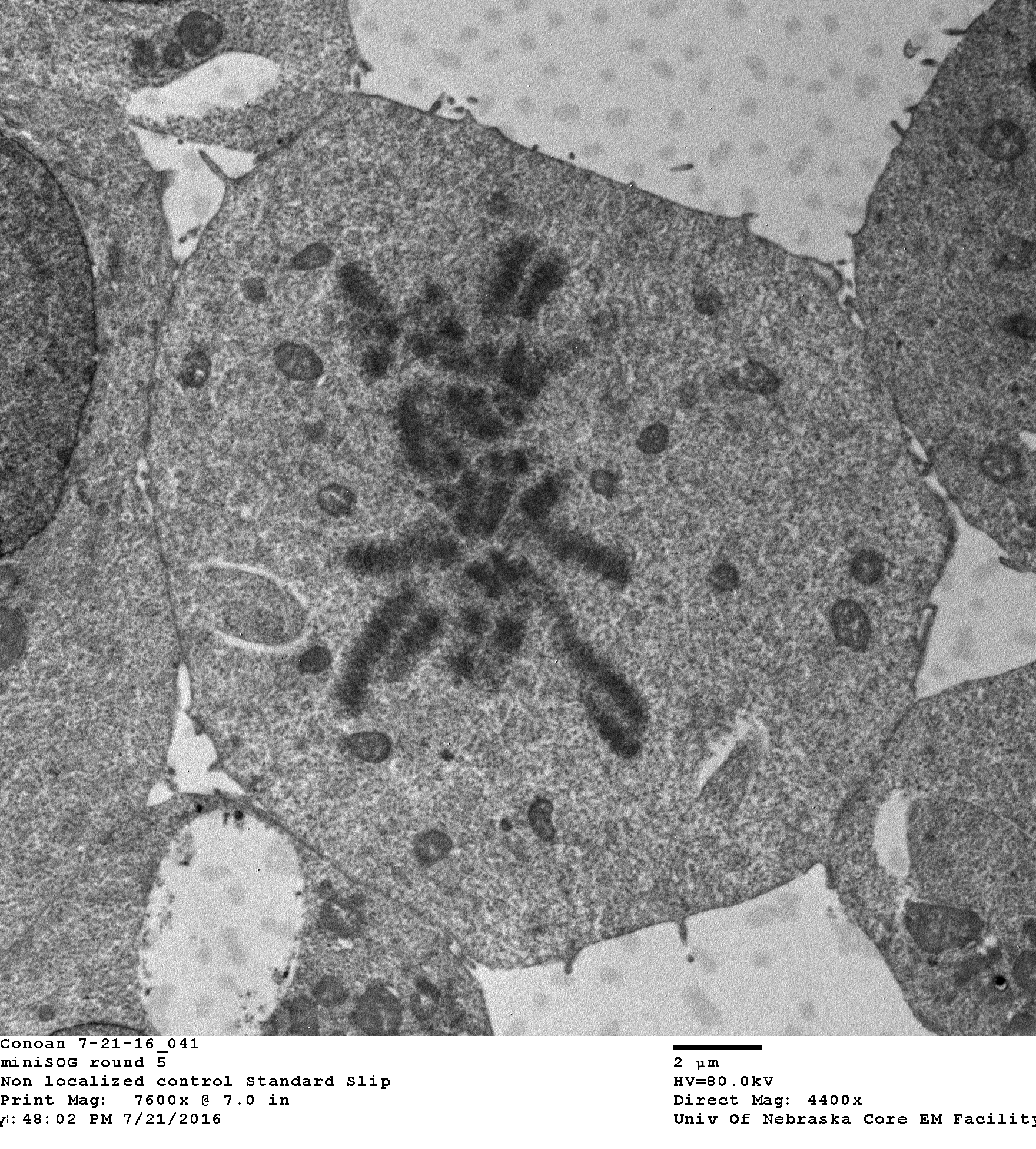This detailed black-and-white photograph, taken through a microscope at the University of Nebraska Core EM Facility, captures a close-up of a small-celled organism labeled with the code NOAN 7-21-16-041. The specimen, identified as "Minisog, round 5," is displayed in a format known as "Non-localized control, standard slip." The print magnification is set at 7600x at 7.0 inches. The photograph records a timestamp of 48 colon 02 PM on July 21, 2016, using an acceleration voltage of 80.0 kV. The direct magnification listed is 4400x. In the center of the image, the oval-shaped cell features numerous dark, small ovals scattered across its surface with a distinctive spider-shaped structure in its middle. Flanking the central cell are partially visible similar cells on either side. The background exhibits a light gray hue dotted with darker gray spots.